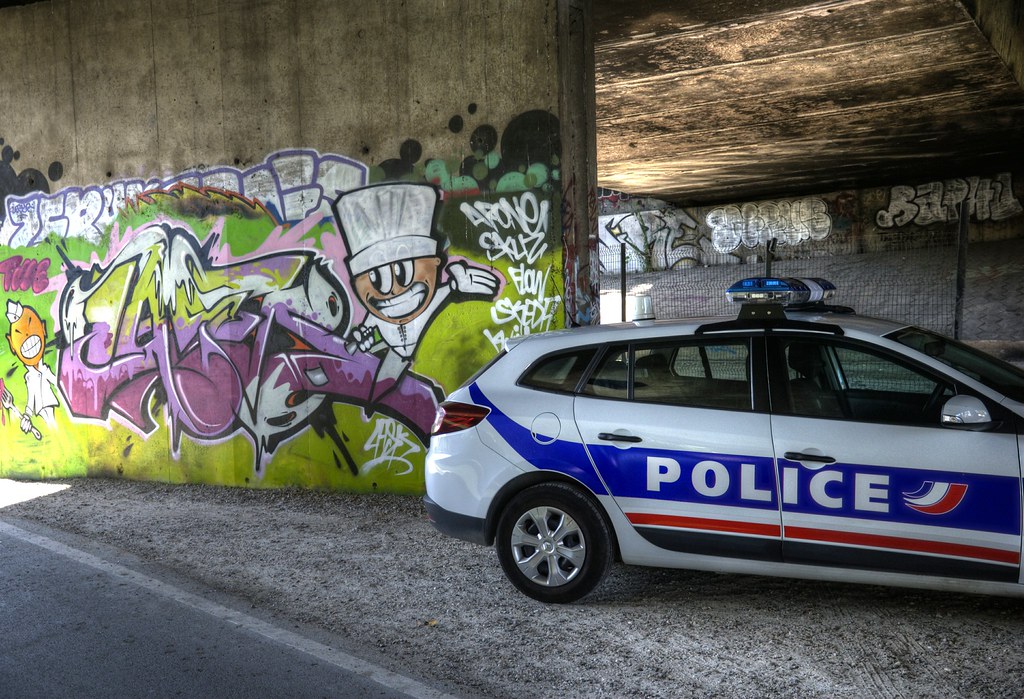The photograph showcases an urban scene taken beneath an overpass, revealing the underside of the roadway supported by cement barriers covered in vibrant graffiti. The graffiti, featuring hues of pink, white, orange, green, and yellow, contains intricate, multi-colored lettering that is difficult to decipher. Dominating the graffiti is a cartoon-like character with a white hat resembling a chef's hat, flashing a wide grin that reveals the whites of its teeth, and waving with a gloved left hand. On the far left, another small figure, wearing a white jacket and a hat shaped like an army corporal's cap, stands out. To the right of the graffiti is a police car, predominantly white with a hatchback design. The vehicle features a blue banner along its side that reads “POLICE” in white letters, with a red stripe and a black stripe running below it along the length of the car. The car is parked facing slightly off-screen to the right, and its visible police light is blue, contributing to the orderly yet colorful urban tableau.